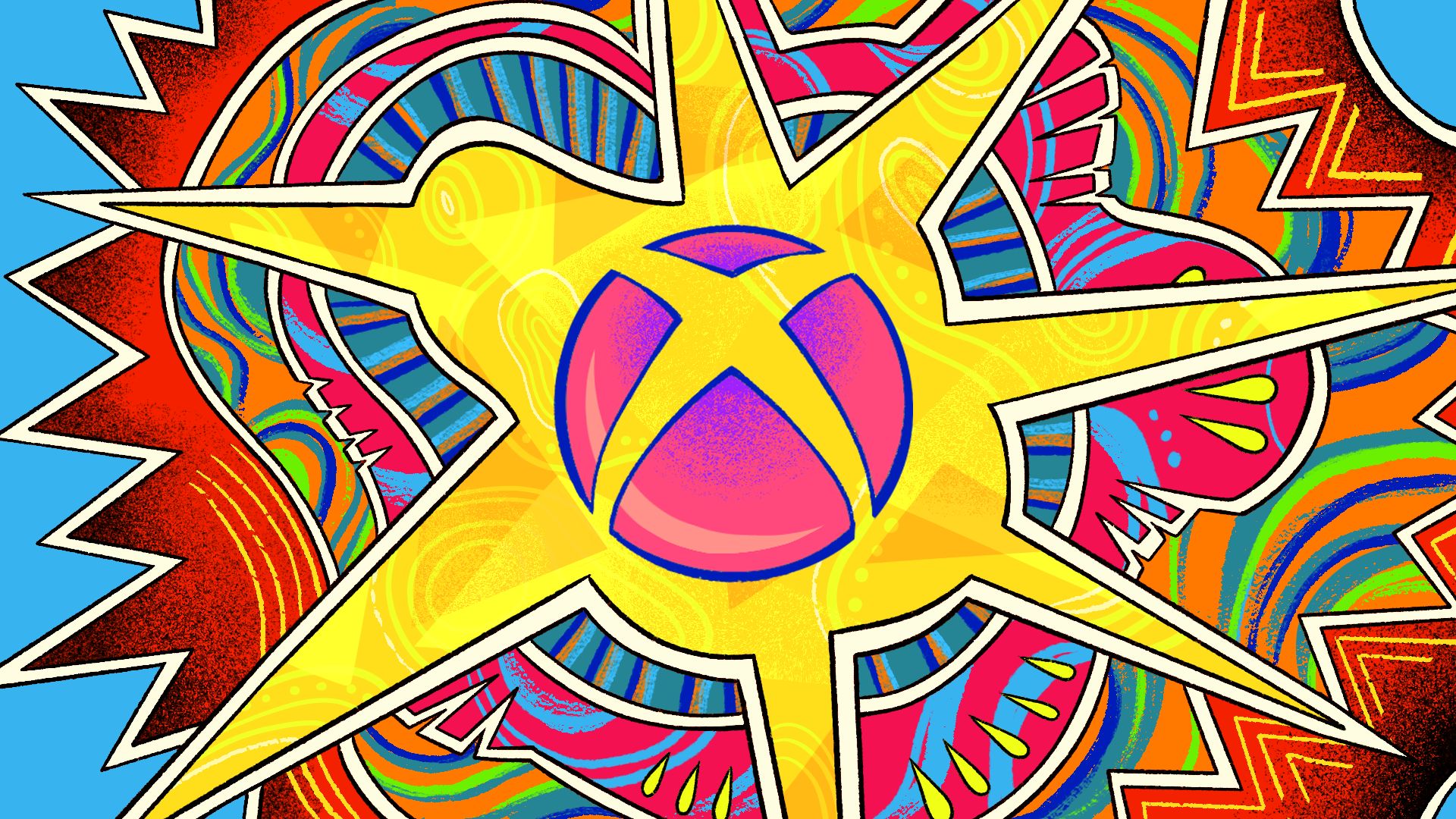The image is a vividly colorful, digitally generated graphic artwork with a blue background. At the heart of the composition lies an intricate, abstract design resembling an organic sun with swirling red spikes, each spike outlined in white. Surrounding this are wavy, multi-colored lines that add dynamic movement to the piece. Central to the image is a star-like shape with yellow and orange patterns that vaguely suggest the form of a bird with a beak. This star is surrounded by additional smaller designs, including teardrop shapes and more swirling patterns in hues of red, green, blue, and orange. In the very center is a spherical shape that transitions from purple to bright pink, featuring a yellow cross at its core and bordered in dark blue. The overall image exudes a sense of dynamic energy and abstract artistry, reminiscent of the vibrant panels in an animated graphic novel.